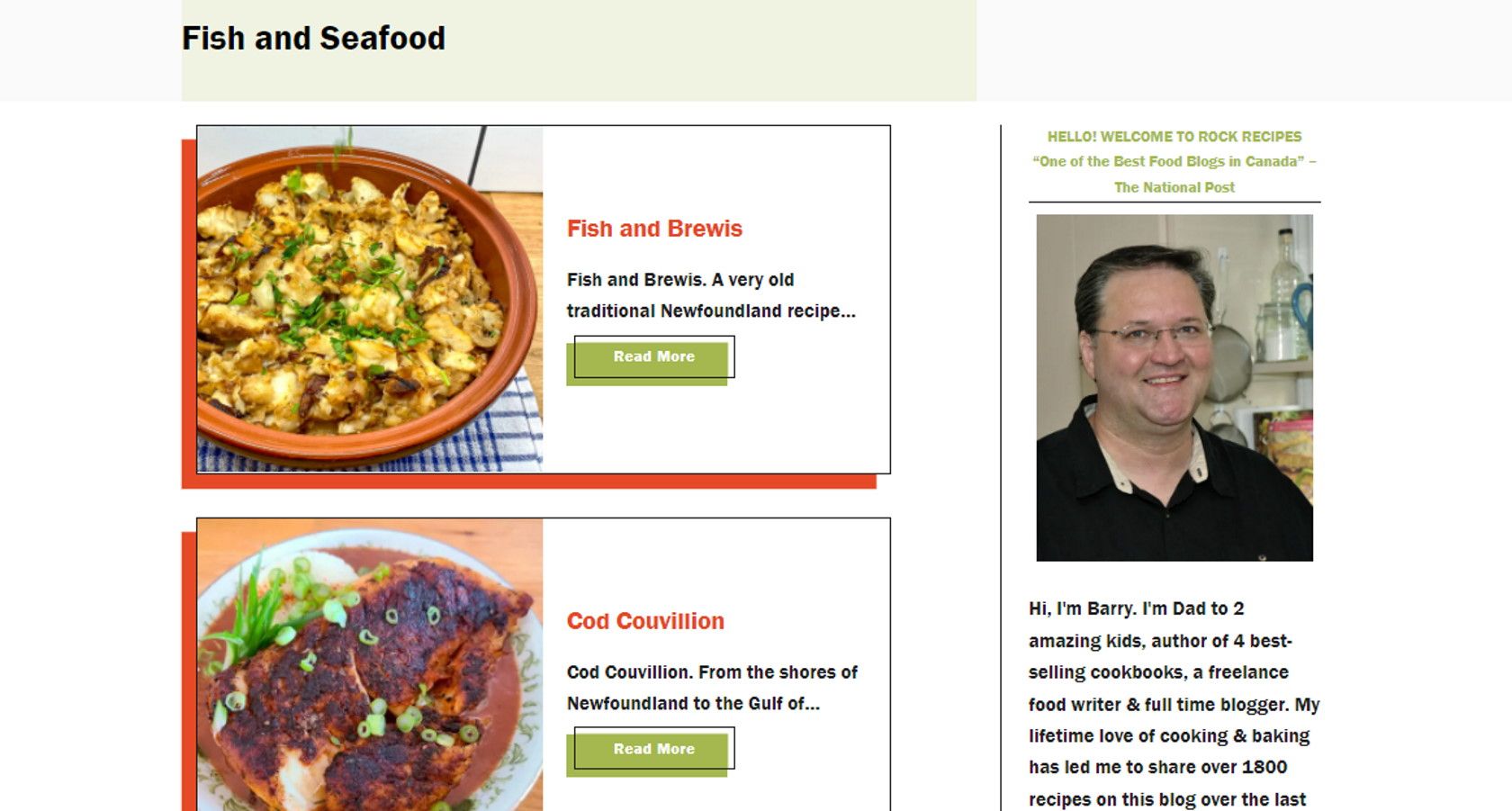This advertisement for Rock Recipes, one of the best food blogs in Canada according to the National Post, features a light green border at the top with "Fish and Seafood" written in black font. Below, there are two images of traditional Newfoundland dishes, each on white backgrounds with black and red borders. The first dish is Fish and Brewis, labeled as a very old traditional Newfoundland recipe, with a green "Read More" link bordered in black. The second dish is Cod Couvillion, described as being from the shores of Newfoundland to the Gulf of... with a similar "Read More" link. To the right of the dishes is a photograph of Barry, the founder of Rock Recipes. The accompanying text in green font reads, "Hello, welcome to Rock Recipes, one of the best food blogs in Canada." Below the photo, black text introduces Barry as the dad to two amazing kids, author of four best-selling cookbooks, a freelance food writer, and a full-time blogger. His love for cooking and baking has resulted in over 1,800 recipes shared on his blog.